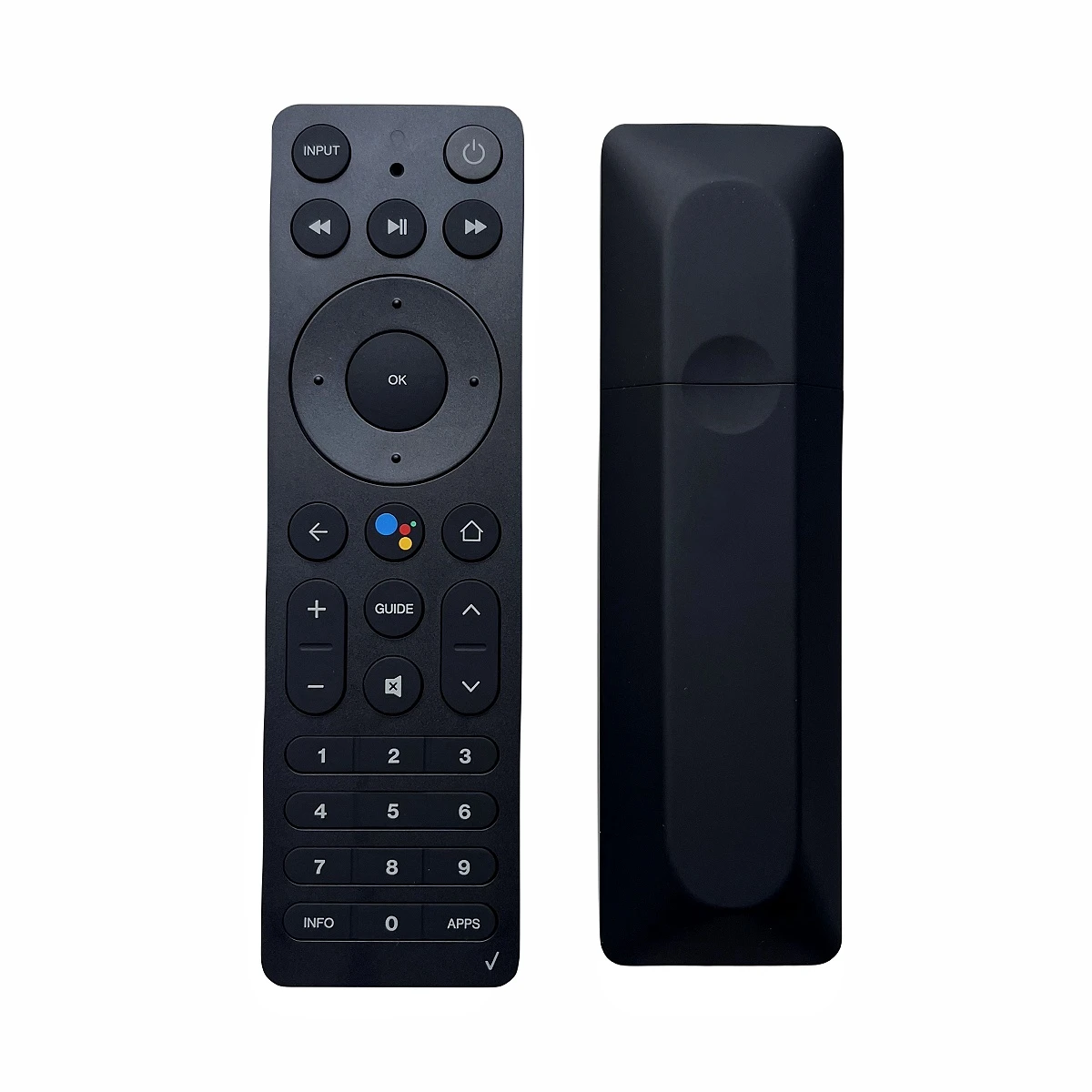This photograph showcases both the front and back views of a solid black remote control against a white background. On the left side, the front of the remote features a detailed array of buttons. At the top, there are two black buttons; the left one is labeled "Input" in white font, and the right one displays the power symbol. Directly below these, three buttons are positioned functionally for rewinding, stopping or pausing, and fast forwarding. The central section hosts a circular directional pad with a prominent "OK" button in the middle, allowing navigation in up, down, left, and right directions. Encircling this pad, there are additional buttons: a left-pointing arrow, a "Home" button, and pill-shaped volume control buttons marked with a plus and minus symbol. Below the directional pad, there's a colorful circular button divided into four quadrants of blue, green, red, and orange, next to which sits another "Home" button. Further down, a standard numeric keypad includes buttons for numbers 1 through 9 and 0, supplemented by additional functional buttons such as "Guide," "Mute," channel switching arrows, "Info," and "Apps." The right side of the photograph displays the back of the remote, continuing the simplistic design.